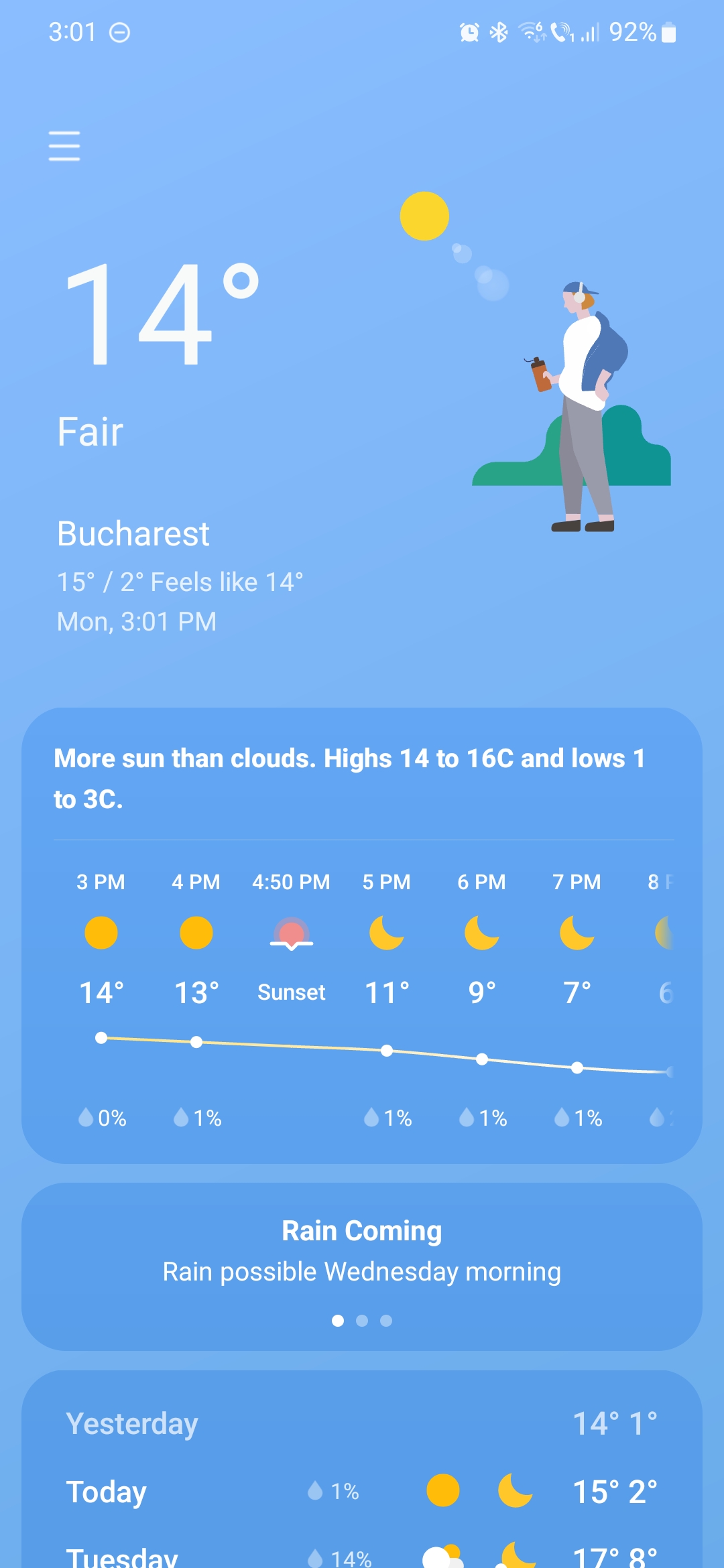This screen capture from a weather app on a smartphone provides a detailed summary of current weather conditions and future forecasts. At the top of the screen, the phone's status bar displays various icons including a driving wheel next to '3:01 PM', an alarm clock, a Bluetooth symbol, internet connectivity, WiFi calling status, signal bars, and battery life showing 92%.

On the app interface, the top left corner has a menu icon (three lines). The main display states that it is 14°C and the weather is fair in Bucharest. Below this, the high for the day is 15°C and the low is 2°C. Additionally, it mentions that it currently feels like 14°C and it is Monday at 3:01 PM. Adjacent to this weather summary, there is an image of a person walking through a park holding a water bottle and wearing headphones.

Further down, the first box on the app provides a short-term weather forecast, indicating "More sun than clouds" with highs between 14-15°C and lows between 1-3°C. It also details the hourly temperature progression: it remains 14°C and then drops to 13°C, with sunset scheduled for 4:50 PM, after which temperatures will continue to decrease.

Below this, there is an alert stating "Rain coming," with a note that rain is possible on Wednesday morning. The bottom section of the screen lists the weather conditions for yesterday (Sunday), today (Monday), and Tuesday, providing a quick glance at past and upcoming weather patterns.